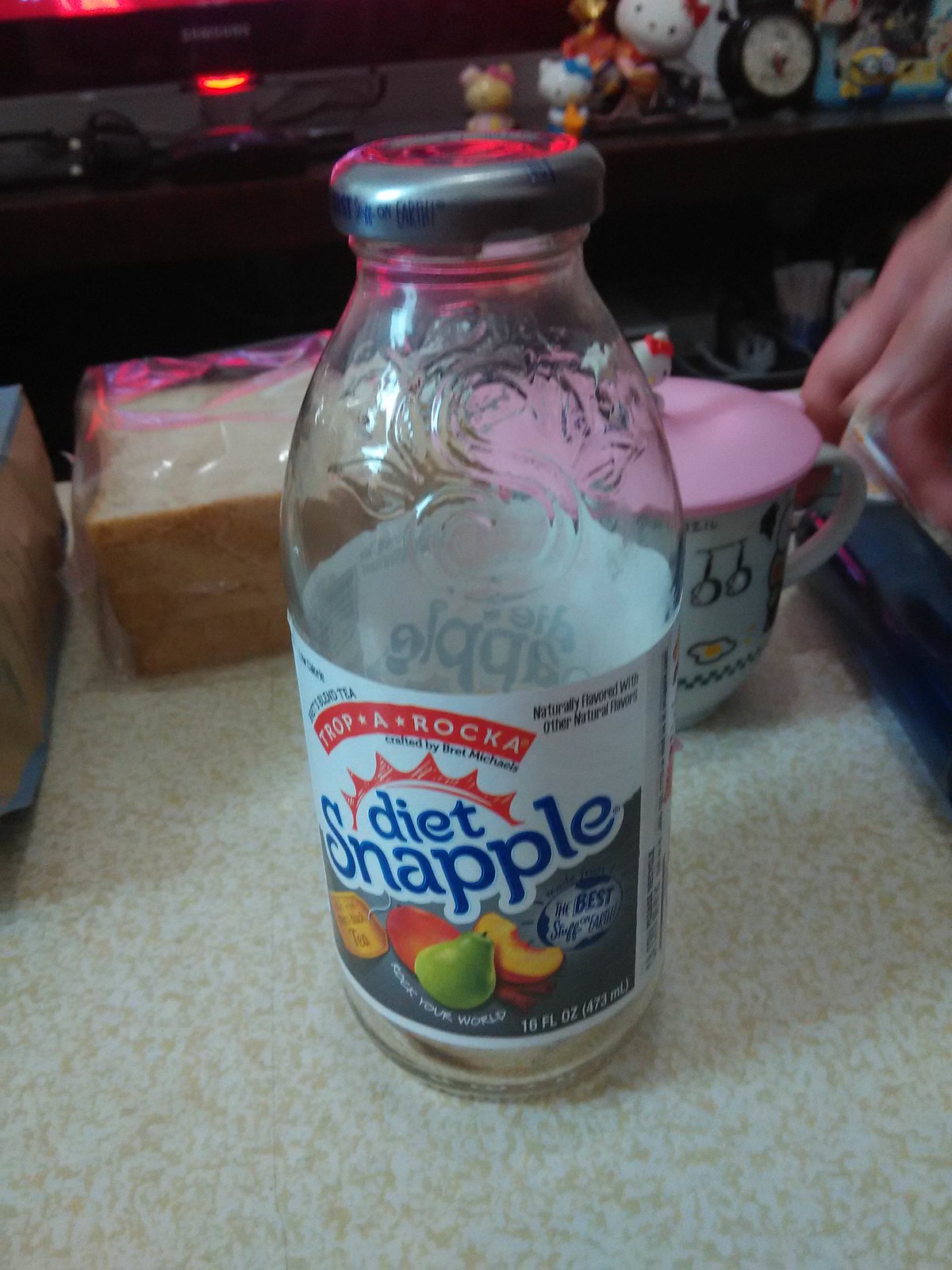The image captures a close-up of a glass Diet Snapple bottle with a silver cap, sitting on a white and beige speckled kitchen countertop. The label on the bottle is detailed with a combination of white, blue, gray, red, and black text and images. Prominently displayed on the label are pictures of a pear, a peach, and a mango or similar orange-red fruit, though some of the text is unclear. The label also includes messages like "TROB ROCKER" in white on a red background, "DIET SNAPPLE" in blue, "Naturally Flavored with Other Natural Flavors," and "Rock Your World." Behind the bottle, there is a plastic-wrapped loaf of white bread, a white coffee cup, and various objects including pots and pans, a Hello Kitty lid with a red bow, and a cap with a yellow yolk image. There's also a hand visible on the right side of the image and a black object beneath it. The scene conveys a regular kitchen setting with everyday items scattered on the countertop.